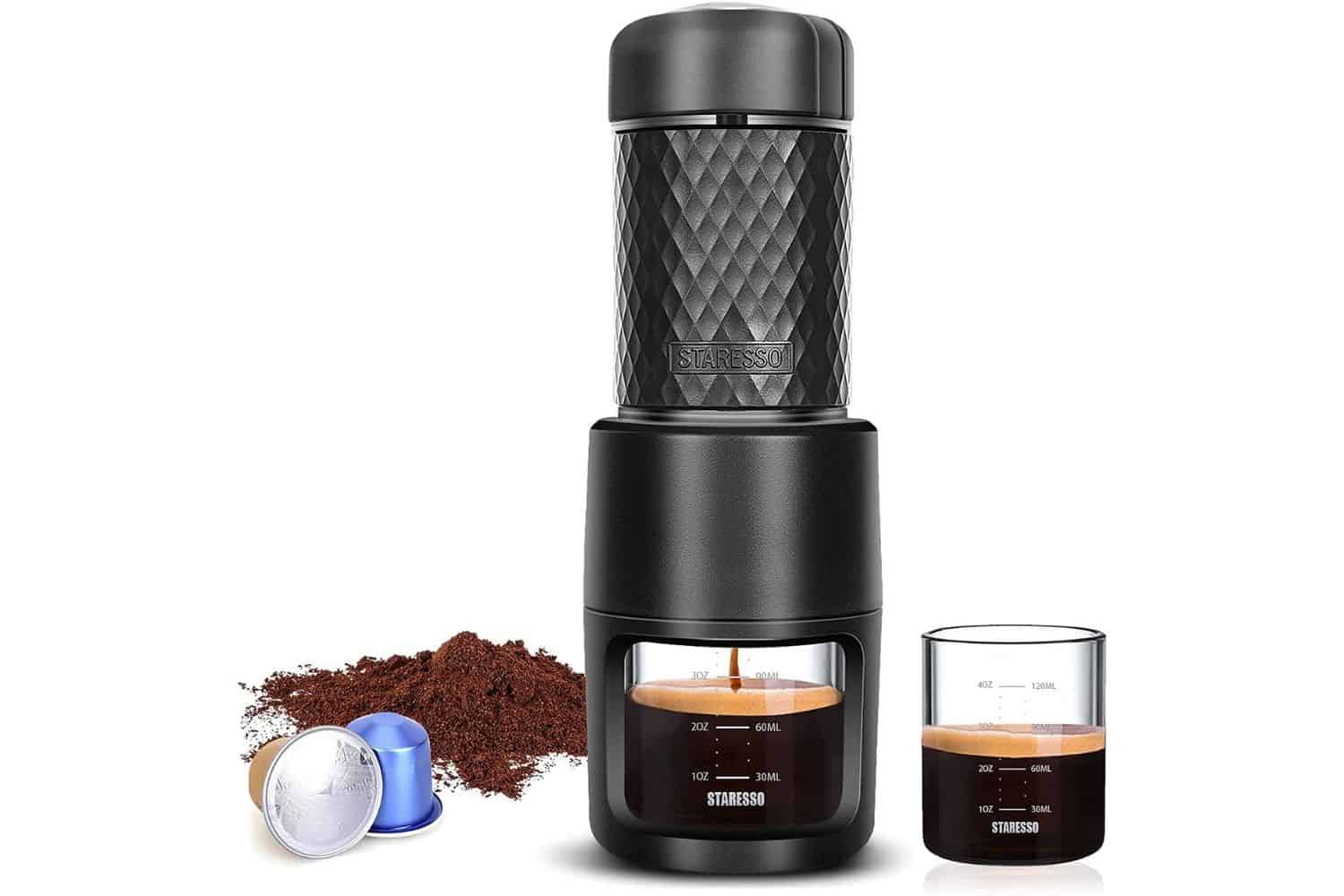The image is a professional advertisement showcasing a sleek, black cylindrical coffee maker by the brand Staresso, standing in front of a white background. The coffeemaker features a smooth black top encircled by a silver ring, followed by a black waffle-patterned cylinder, another silver ring, and a matte black base. It is actively brewing coffee into a clear glass beaker inserted into it. The beaker, marked with the brand name "Staresso" and measurement lines for 1, 2, 3, and 4 ounces, is catching the dark liquid topped with light brown foam. 

To the right of the coffeemaker, a similar beaker with identical measurements, also filled with freshly brewed coffee and foam, is positioned. On the left side of the coffeemaker, there is a mound of black coffee grounds and two reusable or disposable coffee pods with silver tops—one yellow pod lying on its side, and a light purple pod standing upright behind it. The overall composition of the elements in the image, combined with the clean white background, gives it a polished and professional look.